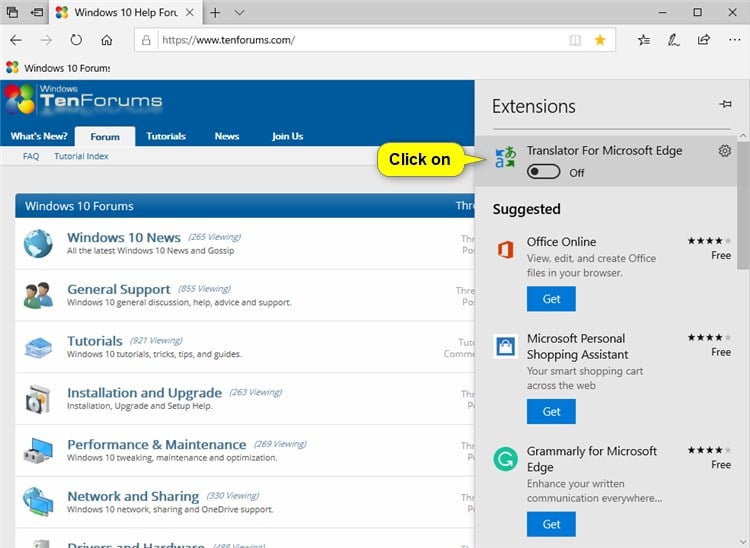The image showcases an old-style Internet website format of a Windows 10 Help Forum. In the upper left-hand corner, there is a tab labeled "Windows 10 Help Forum," accompanied by a Windows-style icon with red, green, blue, and yellow colors. The upper right-hand corner features the typical Minimize, Maximize, and Close (X) buttons. 

Below these, a toolbar hosts a Back arrow, Forward arrow, Refresh button, and Home button. The address bar displays the URL "www.10forums.com" with a yellow star on the right indicating it is favorited. 

A banner in blue reads "Windows 10 Forum," with navigation links for "What's New," "Forum," "Tutorials," "News," and "Join Us." The "Forum" tab is highlighted. The forum sections listed include "Windows 10 Forums," "Windows 10 News," "General Support," "Windows 10 General Discussion," "Help, Advice, or Support," "Windows 10 Tutorials," "Tricks, Tips, and Guides," "Installation and Upgrade," and "Setup Help." Further categories cover "Performance and Maintenance," "Windows 10 Tweaking, Maintenance, and Optimization," and "Network and Sharing," which includes "Windows 10 Network," "Sharing," and "OneDrive Support."

In the upper right-hand corner, there is an "Extensions" menu for Microsoft Edge, showing "Translator for Microsoft Edge" as currently off, with a yellow button labeled "Click On." Suggested extensions include "Office Online," "Microsoft Personal Shopping Assistant," and "Grammarly for Microsoft Edge."